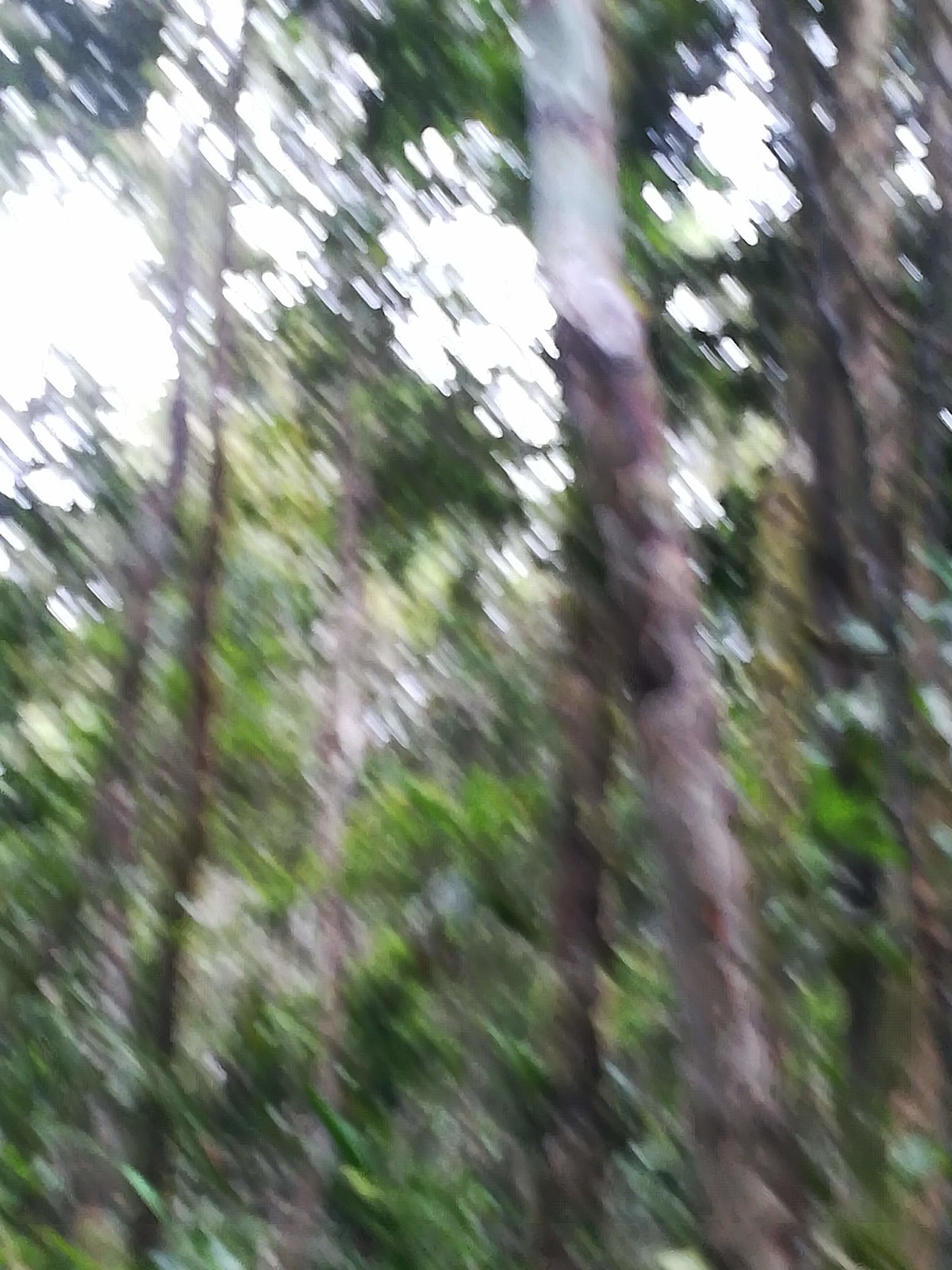The image captures a pair of trees characterized by gray and brown trunks and a mix of light and dark green leaves, with a few brown leaves interspersed. However, the photograph is rendered indistinct due to motion blur, likely caused by the rapid shaking of the camera at the moment the picture was taken. This results in an abstract swirl of colors and shapes, obscuring any fine details and creating a dynamic and somewhat chaotic visual effect.